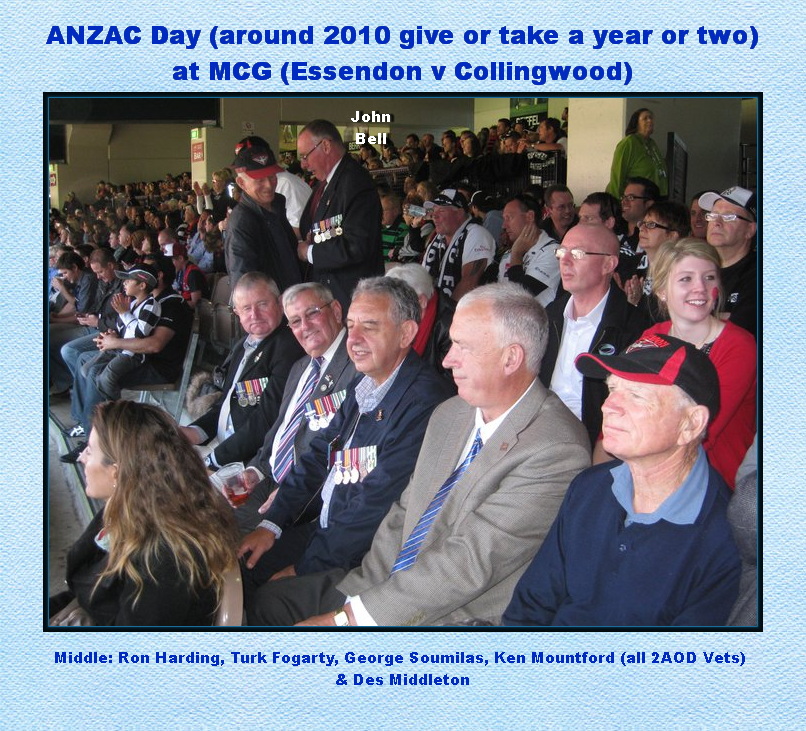The postcard-style image captures the vibrant atmosphere of the ANZAC Day event at the MCG, around 2010, during the Essendon vs. Collingwood match. The card features a blue border with dark blue text at the top, stating: "ANZAC Day (around 2010, give or take a year or two) at MCG (Essendon v. Collingwood)." The focal point of the photograph is a row of distinguished gentlemen, adorned in suits and wearing military medals of honor, indicating their status as veterans. These men are identified at the bottom in blue text as Biddle, Colin, Ron Harding, Turk Fogarty, George Samoulis, Ken Mountford (all 2AODV vets), and Des Middleton.

The scene is animated by a crowded arena of supporters, with several details adding to the lively ambiance. Notably, a girl in the second row has a red face painting, and another girl in the foreground is donning a black jacket. The men appear to be engaged in conversation, smiling and enjoying the event. Among the crowd, a man is seen standing and shaking hands with another man in a black and red cap, who is also wearing a black jacket. This image encapsulates a moment of camaraderie and collective memory, honoring the veterans amidst the bustling excitement of the ANZAC Day match.